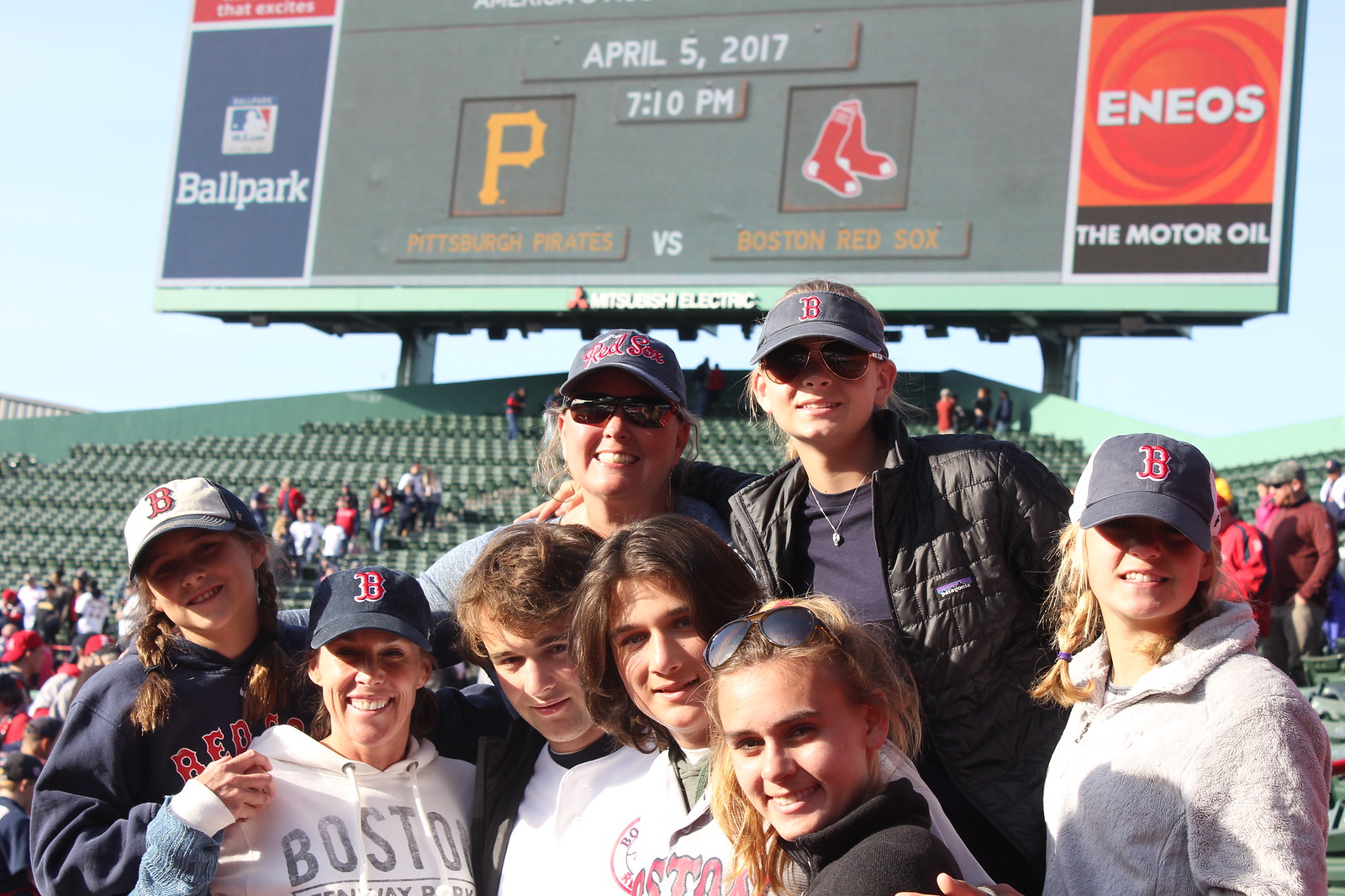Captured at Fenway Park in Boston, this image dates to April 5th, 2017, at 7:10 PM, ahead of a game between the Pittsburgh Pirates and the Boston Red Sox. In the foreground, a group of eight fans—mostly women and possibly two men—poses excitedly for the camera. They sport Boston Red Sox caps, hoodies, jackets, and sunglasses, suggesting chilly weather. Behind them, stadium seats are visible with a scattering of seated attendees. A large scoreboard looms above, displaying the game details with branding for "Ballpark," "Eneos the Motor Oil," and "Mitsubishi Electric," amidst a backdrop of partially filled stands.